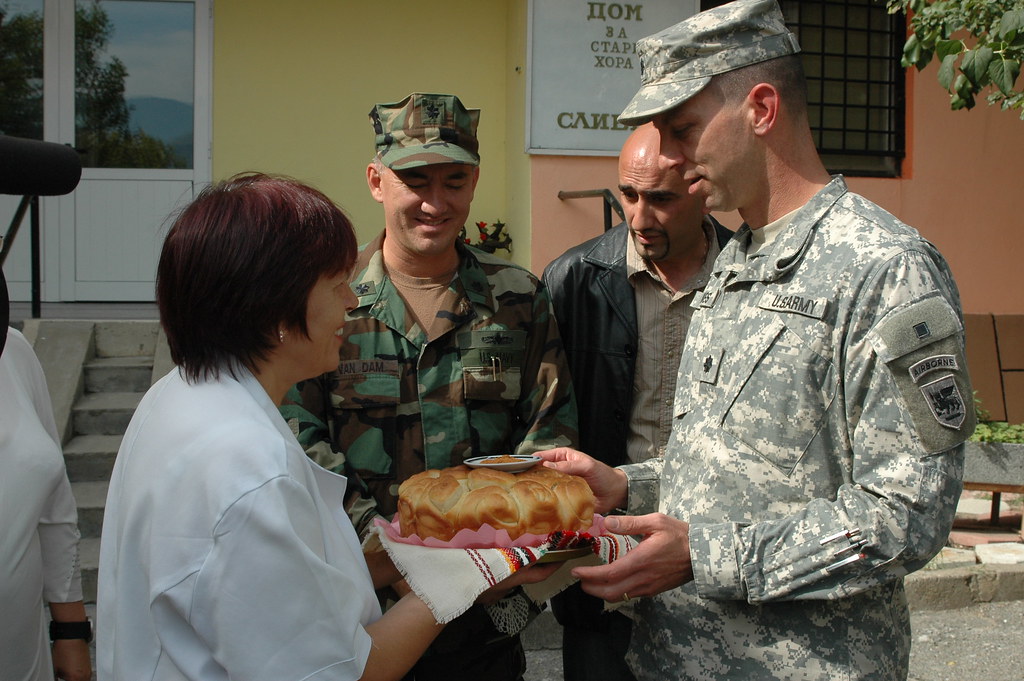The image captures an outdoor scene in bright daylight, featuring a group of four central figures. A woman with short dark hair, dressed in a white short-sleeved shirt, stands to the left holding a circular brown bread on a plate, covered with a white towel with brown stripes, and topped with a small, hard-to-see orange-filled bowl. In front of her, a white male soldier dressed in a green camouflage U.S. Army uniform with a cap and shoulder patches, looks at the food. Next to him is another soldier in a darker camouflage outfit. A bald civilian man with a goatee stands between the soldiers, wearing a black leather jacket over a light gray button-down shirt. The background shows a building with a smooth concrete façade, half painted in yellow and half in light pink, possibly featuring some Asian script. There is ample lighting, providing a clear view of the scene, and shadows are cast on the street, suggesting a sunny day.